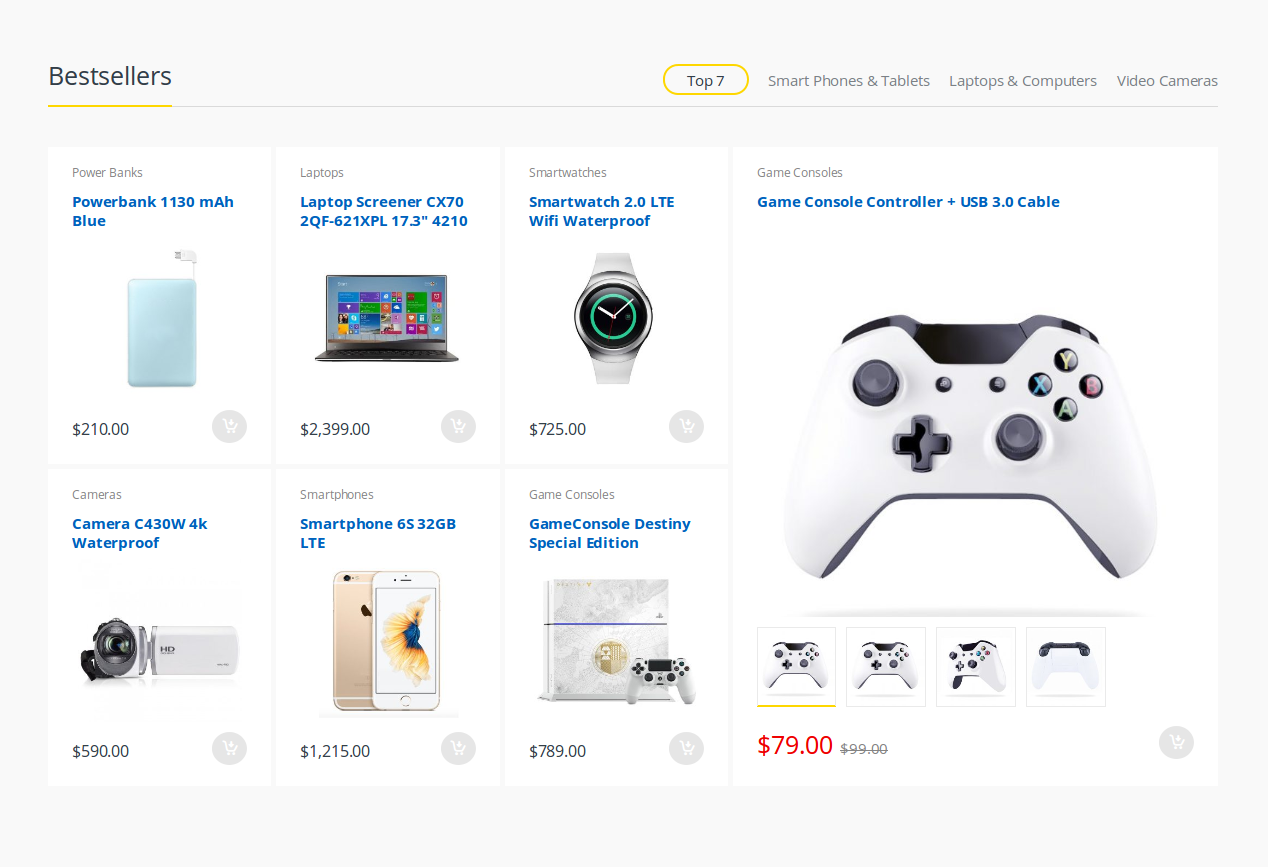**Caption:**

The image features a shaded gray square with the text "Best Sellers" in black on the left side, accompanied by a small yellow line underneath it. At the center, the text "Top Seven" appears in black, surrounded by a yellow circle. Below this header, three categories are listed in gray: "Smart Phones and Tablets," "Laptops and Computers," and "Video Cameras."

Displayed beneath the categories, the image showcases a selection of product images: three on the top row, three on the bottom row, and one prominent image on the right. The descriptions and details of each product are as follows:

1. **Power Banks**:
   - **Description**: Power Bank, 1130MAH, Blue
   - **Image**: A blue power bank
   - **Price**: $210

2. **Laptops**:
   - **Description**: Laptop Screen or CX70, 17.3 inch
   - **Image**: A laptop
   - **Price**: $2,399

3. **Smart Watches**:
   - **Description**: Smart Watch, 2.0 LTE Wi-Fi Waterproof
   - **Price**: $725

4. **Cameras** (Bottom left):
   - **Description**: Camera, C430W 4K Waterproof
   - **Image**: A camera
   - **Price**: $590

5. **Smart Phones**:
   - **Description**: Smart Phone, 6532GB LTE
   - **Image**: A white smartphone
   - **Price**: $1,215

6. **Game Consoles**:
   - **Description**: Game Console, Destiny Special Edition
   - **Price**: $789

7. **Main Feature (Right side)**:
   - **Description**: Game Console Controller with USB 3.0 Cable
   - **Image**: A white device with buttons
   - **Additional Details**: Includes four smaller images beneath it
   - **Pricing**: Originally $99, now discounted to $79 (marked in red with the original price crossed out)